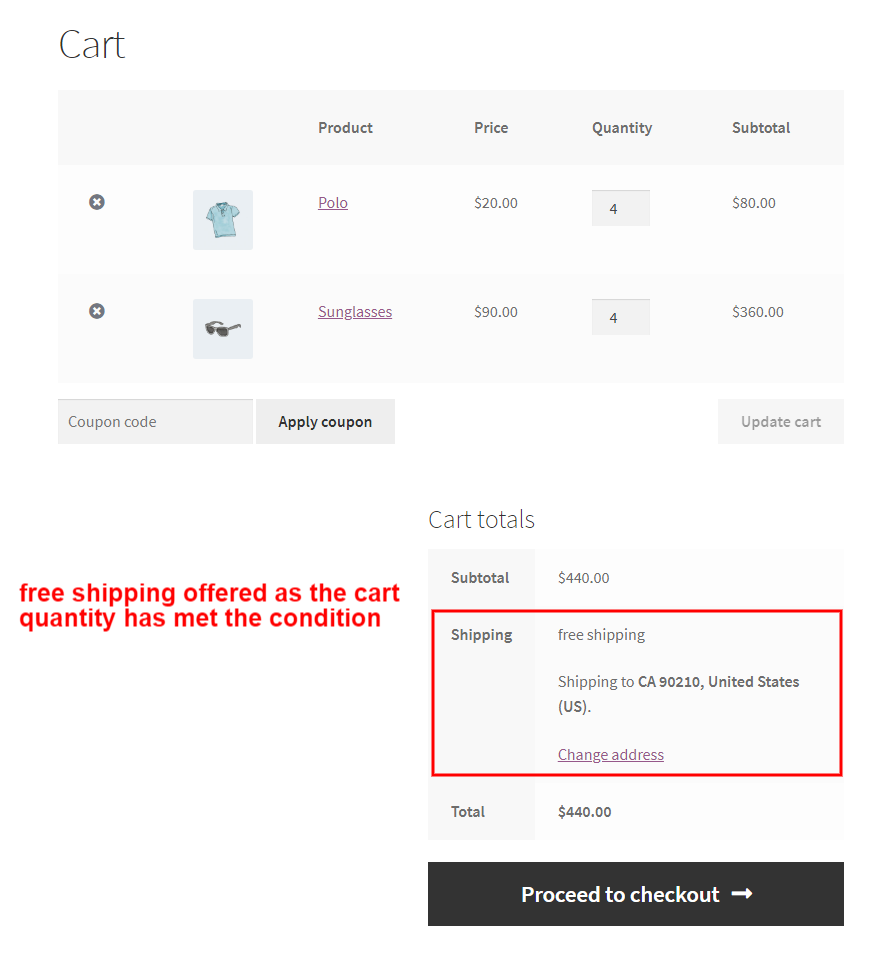A detailed printout of an online shopping cart displays a summary of items selected for purchase. At the top, the title "Cart" is prominently shown. Below this, a header row contains the labels "Product," "Price," "Quantity," and "Subtotal" from left to right. The first item listed is a blue polo shirt, accompanied by a thumbnail image. It is priced at $20 each with a quantity of 4, making the subtotal $80. The second item is a pair of sunglasses, also with an image beside it. Each pair is priced at $90 and the quantity is 4, totaling $360. Beneath the itemized list, clickable options labeled "Coupon Code," "Apply Coupon," "Update Cart," and "Cart Options" are available. Following this, the "Cart Totals" section is detailed. In red text, it mentions that free shipping is offered because the cart quantity condition has been met. The subtotal is listed as $440. Enclosed in a red box, the shipping details indicate "Free Shipping" to California, zip code 90210, USA. A "Change Address" option appears just below this. Outside the red box, the total amount of $440 is reiterated, and a black box beneath it contains the "Proceed to Checkout" button, highlighted with a right-pointing arrow in white.